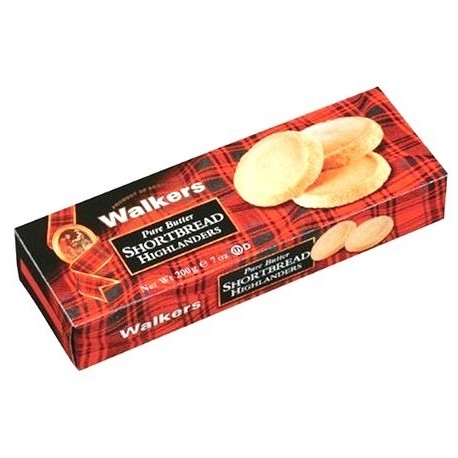The image depicts a rectangular box of shortbread biscuits with a distinctive red and black checker pattern. The box appears against a solid white background. On the top of the box, towards the right, there are three golden yellow shortbread biscuits arranged in a slightly overlapping manner. To the left, the brand name "Walkers" is prominently displayed in white lettering. Below the brand name, there's a black rectangular box containing the words "Pure Butter Shortbread Highlanders" in white. 

An oval image on the top left corner of the box shows two people facing each other, adding a unique visual element. Along the front edge of the box, the left side repeats the brand name "Walkers," followed by another black rectangular box with the same white text "Pure Butter Shortbread Highlanders," and on the far right, there are images of two more shortbread biscuits. Additional text indicates the net weight as 200 grams (7 ounces).

The box design combines elements of traditional Scottish plaid with a modern presentation, giving it an eye-catching and appetizing appearance.